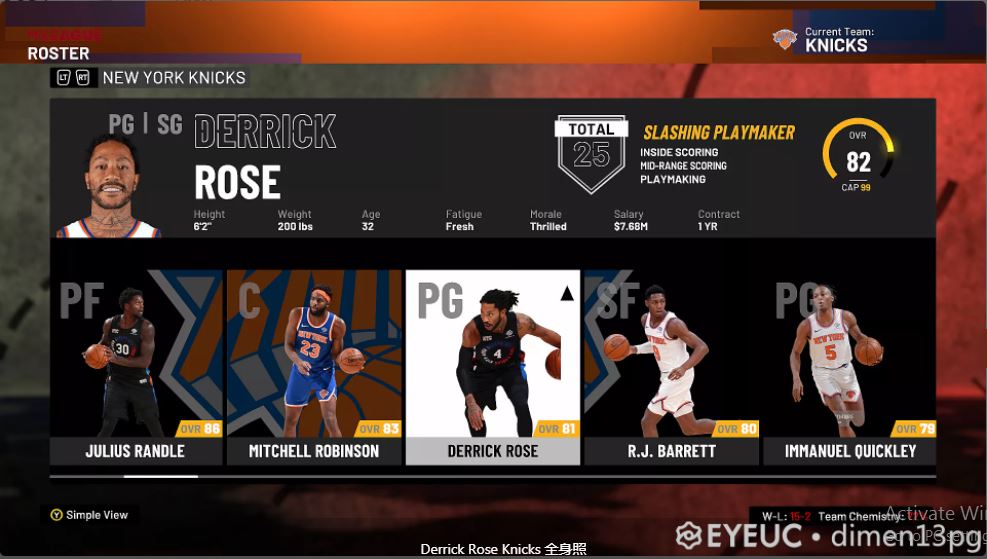This is a horizontal, rectangular image with a dynamic background featuring a blend of oranges, reds, and blacks. Superimposed on this backdrop is another horizontal rectangle which serves as the focal point. The top third of the superimposed image is a gradient light black, where the text "NEW YORK KNICKS" is prominently displayed in bold, all-capital, white font. Above this text, the word "ROSTER" is visible, also in bold, all-capital, white font.

Below this section, the image showcases detailed player information. Next to a photograph of the player, who has a beard, mustache, and is wearing a tank top, the name "DEREK ROSE" is displayed. "DEREK" is in block letters with white outline over a black background, while "ROSE" is in all-capital, white bold font.

To the right of the player’s photo, there is a badge marked with "TOTAL" at the top and the number "25" underneath. Below it, "SLASHING PLAYMAKER" is highlighted in yellow. Three lines of white text list the player's attributes: "Inside Scoring," "Mid-Range Scoring," and "Playmaking." Adjacent to these lines is a semicircle graph, filled about two-thirds in yellow, with the number "82" in the center.

Further down, under Derek Rose's name, additional statistics are outlined with the categories in regular white font and the corresponding data in bold white font. These details include:
- Height: 6 feet 2 inches
- Weight: 200 pounds
- Age: 32
- Fatigue: Fresh
- Morale: Thrilled
- Salary: 7.6M
- Contract: One Year

Beneath these details, vertical images of other players in basketball uniforms with a ball are displayed. These players are Julius Randle, Mitchell Robinson, RJ Barrett (R. J. Barrett), and Immanuel Quickley. Derek Rose’s image is highlighted in white, indicating the focus on him.

At the bottom right corner, the image is labeled with a logo and the text "I-E-Y-E-U-C dot Demen 13-P-J" in all caps.